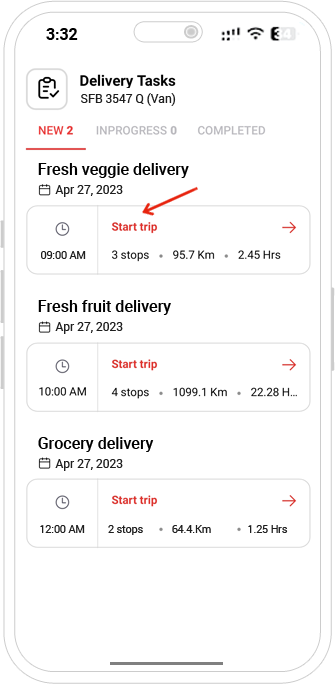This image, taken from a cell phone screen, displays a delivery task interface. At the top of the screen, the section titled "Delivery Tasks" highlights various tasks. The word "New" is prominently marked in red, accompanied by a status bar showing zero tasks "In Progress" and no indication for "Completed" tasks.

Below, under "New," there is an entry for "Fresh Veggie Delivery," scheduled for April 27th, 2023, at 9:00 AM. Next to this entry, a red arrow points downward to a "Start Trip" button, which appears to have been digitally added, likely for instructional purposes. 

Further down, the screen lists additional delivery tasks, such as "Fresh Fruit Delivery" scheduled for 10:00 AM and "Grocery Delivery" set for 12:00 PM. These entries provide a clear breakdown of a delivery schedule, demonstrating appointments and their respective times.